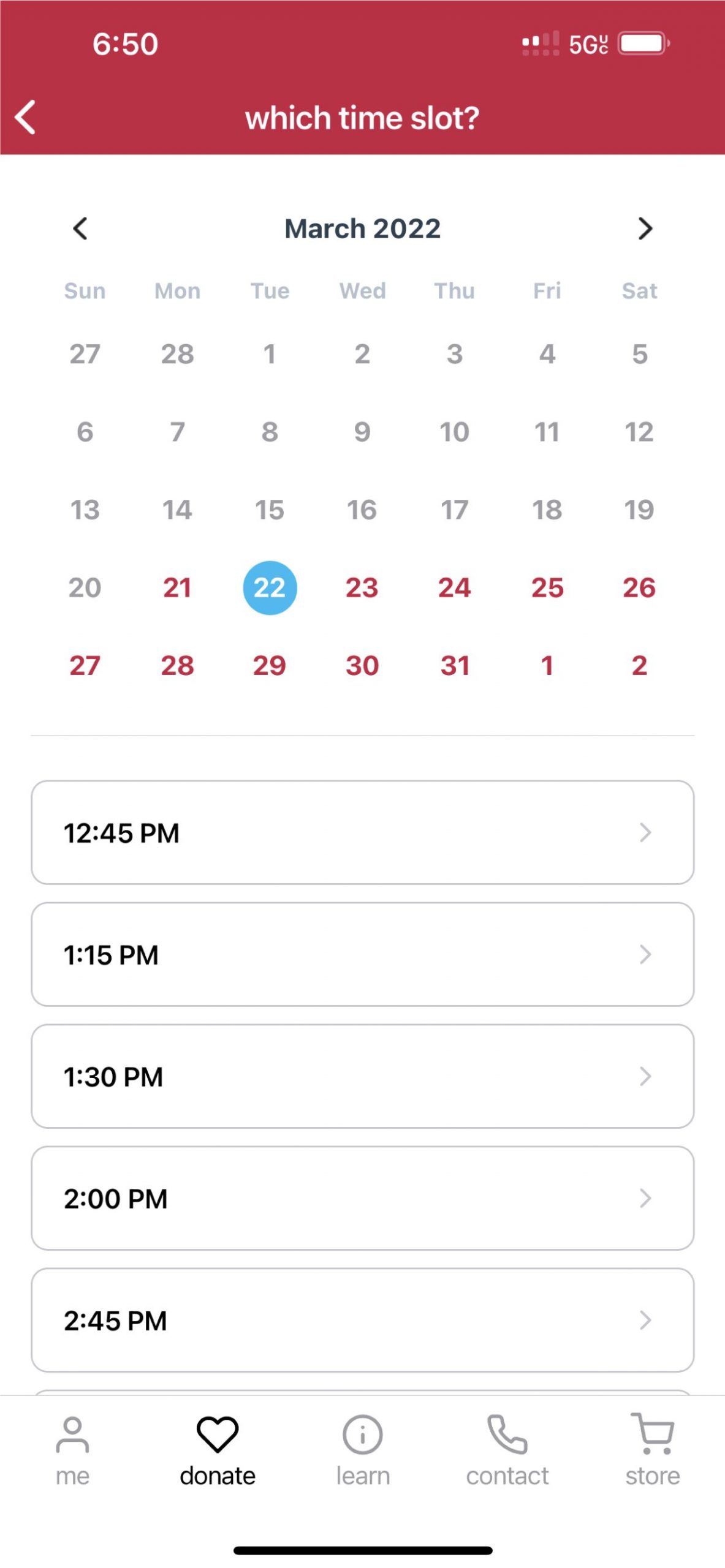The image is a smartphone screenshot with a predominantly burgundy header. At the top left, it displays the number "650" with a left-pointing arrow beneath it. On the top right, the screen indicates a strong 5G signal with full battery life, and only two bars of signal remaining. 

Below the header, on a white background, the text "March 2022" is centered with navigation arrows on either side, allowing the user to switch between months. A week view follows, displaying days in a row from Sunday to Saturday. 

The calendar section starts from February 27-28 at the top left corner, continuing with numbers 1 through 31 for the days of March and ending with April 1-2 on the last two calendar days. A light gray line underlines the calendar.

Beneath this, there are several rectangular-shaped boxes indicating different time slots for appointments or events. The times listed are as follows:

- 12:45 PM
- 1:15 PM
- 1:30 PM
- 2:00 PM
- 2:45 PM